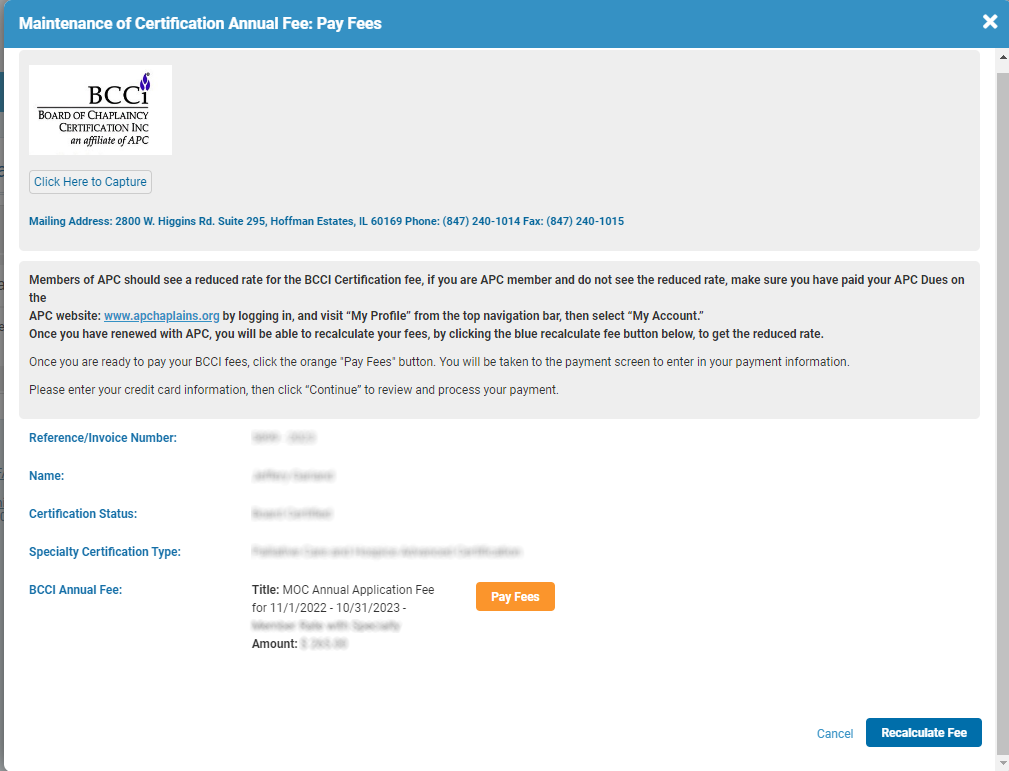The image depicts a detailed webpage from the Board of Chaplaincy Certification Incorporated (BCCI), which outlines the process for maintaining annual certification as a chaplain. At the top, there is a prominent blue bar with the text "Maintenance of Certification Annual Fee" and instructions to "pay fees," along with a link to capture the mailing address provided in Illinois.

The page notes that members of the Association of Professional Chaplains (APC) should see a reduced rate for the BCCI certification fee. It advises APC members who do not see this reduced rate to ensure their APC dues are paid by logging in to the APC website. Specifically, members are instructed to log in, navigate to "My Profile" from the top navigation bar, and then select "My Account."

The webpage suggests that after renewing their APC membership, users can recalculate their fees by clicking the blue "Recalculate Fee" button to see the reduced rate. Once ready to pay the BCCI fees, users should click the orange "Pay Fees" button. This action redirects them to a payment screen where they must enter their credit card information and click "Continue" to review and process the payment.

Below these instructions is a section where multiple fields are grayed out, including reference invoice number, name, certification status, specialty certification type, and the BCCI annual fee. The title "MOC annual" is also mentioned, referring to the annual application fee for the period from November 1, 2022, to October 31, 2023. The exact amount is obscured but is indicated to be at least three digits.